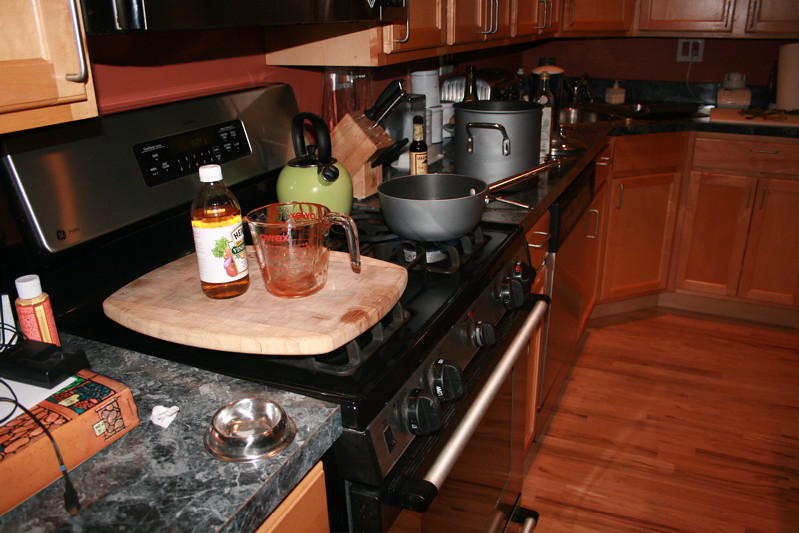This image features a cozy kitchen with a warm and inviting ambiance. The kitchen cabinets are made of rich cherry-colored wood, complemented by sleek gold or silver hardware on the handles. The floor shares the same cherry wood tone, creating a harmonious and cohesive look. The countertops are a striking green marble, adding a touch of elegance to the space.

Black appliances are prominently featured, including a black gas oven and stove, with a matching black microwave mounted above. The stove is in active use, showcasing a black pot and a green kettle with a black handle. A wooden cutting board rests on the stove, holding a measuring cup and a clear bottle with a brownish liquid, suggesting the preparation of a meal.

The walls are painted in a warm terracotta color, enhancing the overall cozy atmosphere of the kitchen. Despite the absence of a backsplash, the wall color adds a rich, earthy feel to the space. On the left side of the counter sits a silver dish, which appears to be an ashtray. In the bottom right corner of the image, there's a glimpse of stacked items including a charging cable and what seems to be a board game or a box.

A large black soup pot can also be seen on the counter in the background, further indicating that this kitchen is actively used and well-loved. This detailed setup not only highlights the functionality of the space but also reflects the personality of its owner.